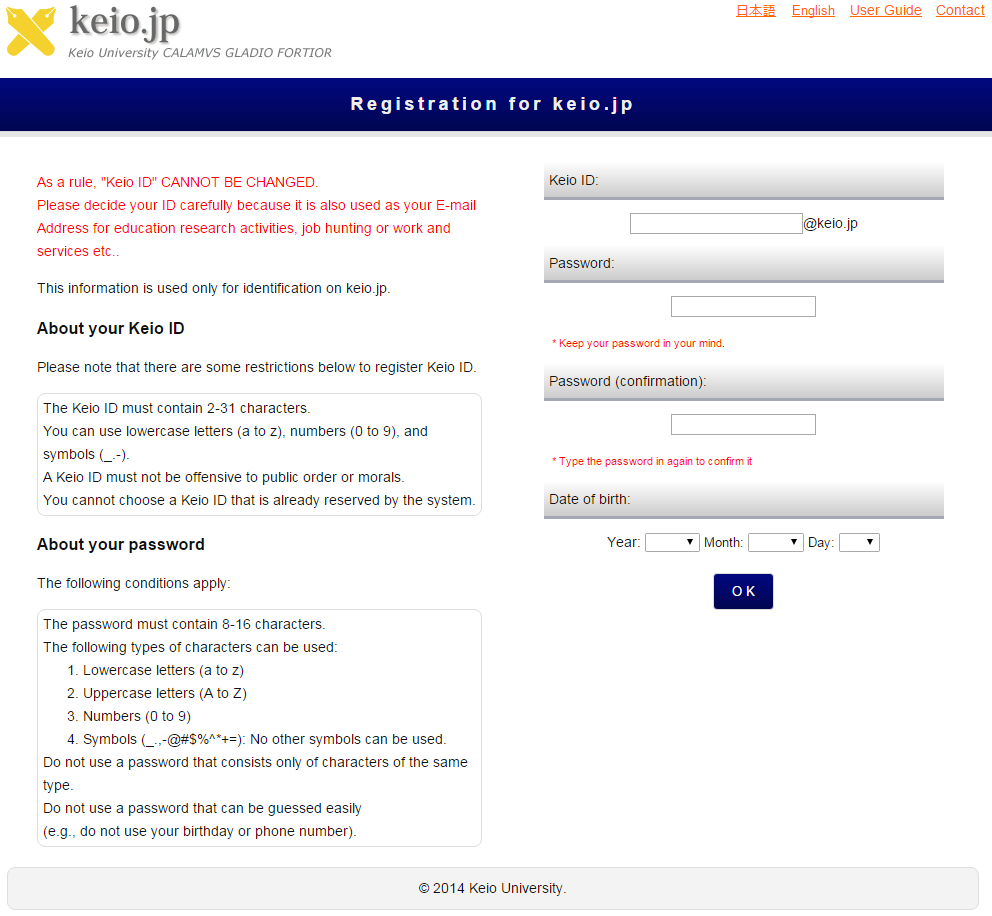The image captures the homepage of the Keio University website (keo.jp). Dominating the top part of the page are the words "Kellogg University" followed by the motto "SCALLAMBS Gladio Fortior." In the upper right-hand corner, there are four navigation options: one in Asian script, "English," "User Guide," and "Contact," all underlined and displayed in an orange font.

Below the navigation options, a long rectangular banner reads "Registration for keo.jp," centered on the page. Underneath this banner, aligned to the left in red font, is a warning stating, "As a rule, Keio ID cannot be changed," followed by additional information in red text.

The next section explains the Keio ID further, featuring a descriptive sentence and a box detailing password requirements, with a heading, "The following conditions apply."

To the right of this section is a form that includes fields for Keio ID, password, password confirmation, and date of birth, culminating with an "OK" button for submission.